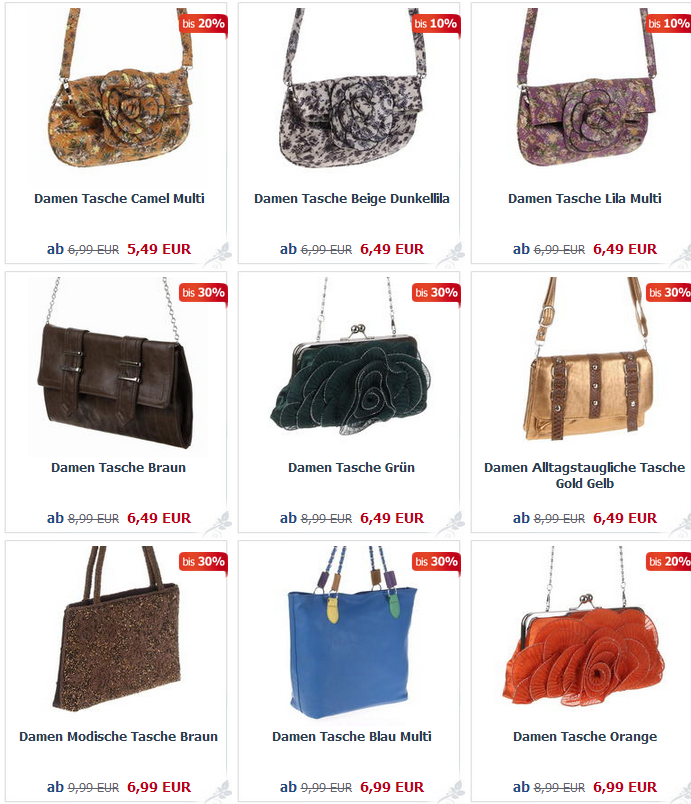The image is a screenshot from a retailer's website featuring nine different handbags, arranged in a 3x3 grid on a white background. Each handbag's name and price are listed in German, with original euro prices crossed out and replaced by red sale prices, indicating discounts ranging from 10% to 30%. 

The top row showcases a single style of purse available in three distinct colors, each adorned with a large floral design made of the same fabric as the purse. The discount varies, with one purse marked at 20% off and the others at 10% off. 

In the middle row, the first handbag is a brown leather-look purse with two buckles and a thin chain handle, labeled as 'Damantasche Braun' and discounted at 30% off. The second, 'Damantasche Grün', is a black purse with a kiss lock clasp and a similar floral design to those in the top row. The third purse in this row, 'Damantasche Gold Gelb', is a messenger bag style, also at 30% off.

The bottom row features three different styles: a plain tote bag in brown, another similar tote bag in blue that appears quite sleek, and a final purse with a kiss lock clasp and floral design similar to others, but in red. All these handbags have labels indicating they are also on sale.

The purse colors range widely including brown, gray, rosy brown, black, green, gold, blue, and red, showcasing a mix of plain and floral designs.